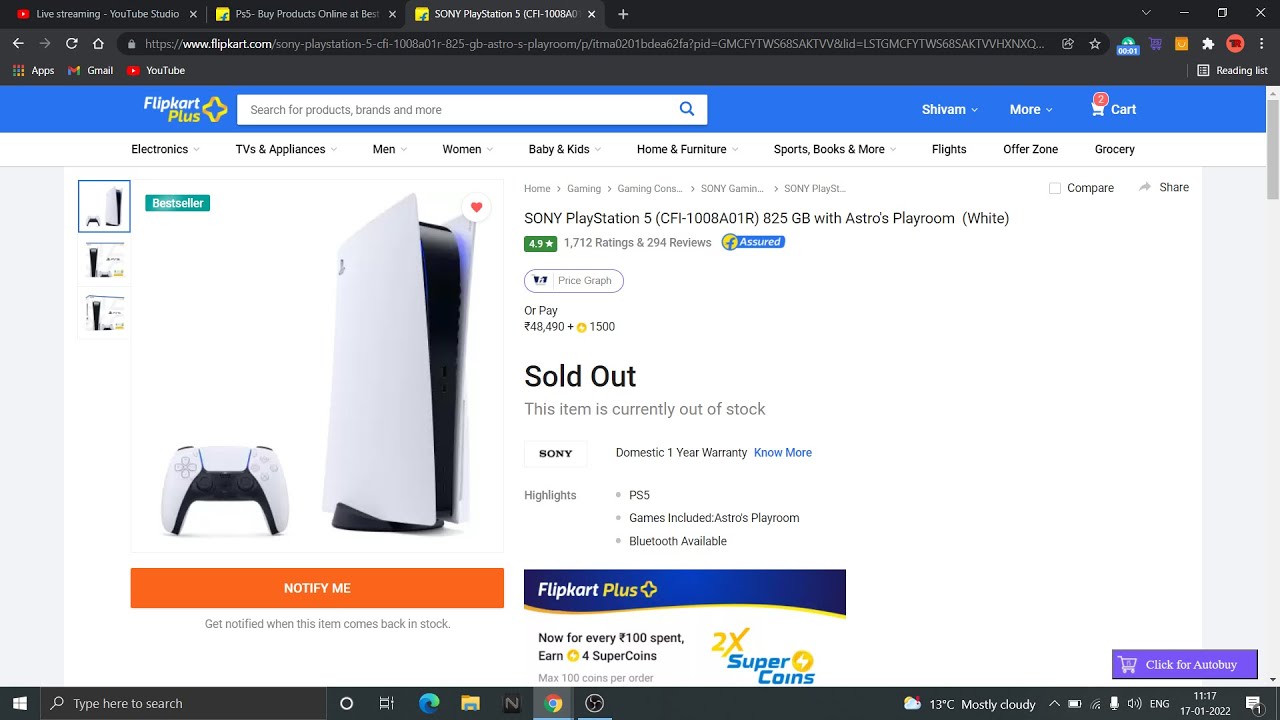A detailed screenshot of a computer screen shows a user on the Flipkart Plus website. The top portion of the image reveals typical browser elements: a black header area containing the Flipkart Plus logo, along with three open tabs. One tab is used for live streaming on YouTube, another for the Flipkart website itself, where the user is shopping for a PlayStation.

Prominently, the middle section of the screen displays a high-resolution image of a Sony PlayStation 5 console with a matching controller on the left side. To the right of the image, detailed product information is presented. The item is identified as a "Sony PlayStation 5, 825GB with Astro's Playroom - White." This product boasts a stellar rating of 4.9 stars based on 294 reviews. Unfortunately, the product is marked as sold out.

At the top of the screen, a search bar is situated alongside an icon of a shopping cart with a number "2" indicating two items within. Below the product description, the right side of the screen features an option labeled "Click for Auto-Buy," while the bottom left highlights an orange "Notify Me" button, allowing users to receive alerts when the product restocks. The layout and details provide a comprehensive glance at the user's current online shopping experience for a highly sought-after console.